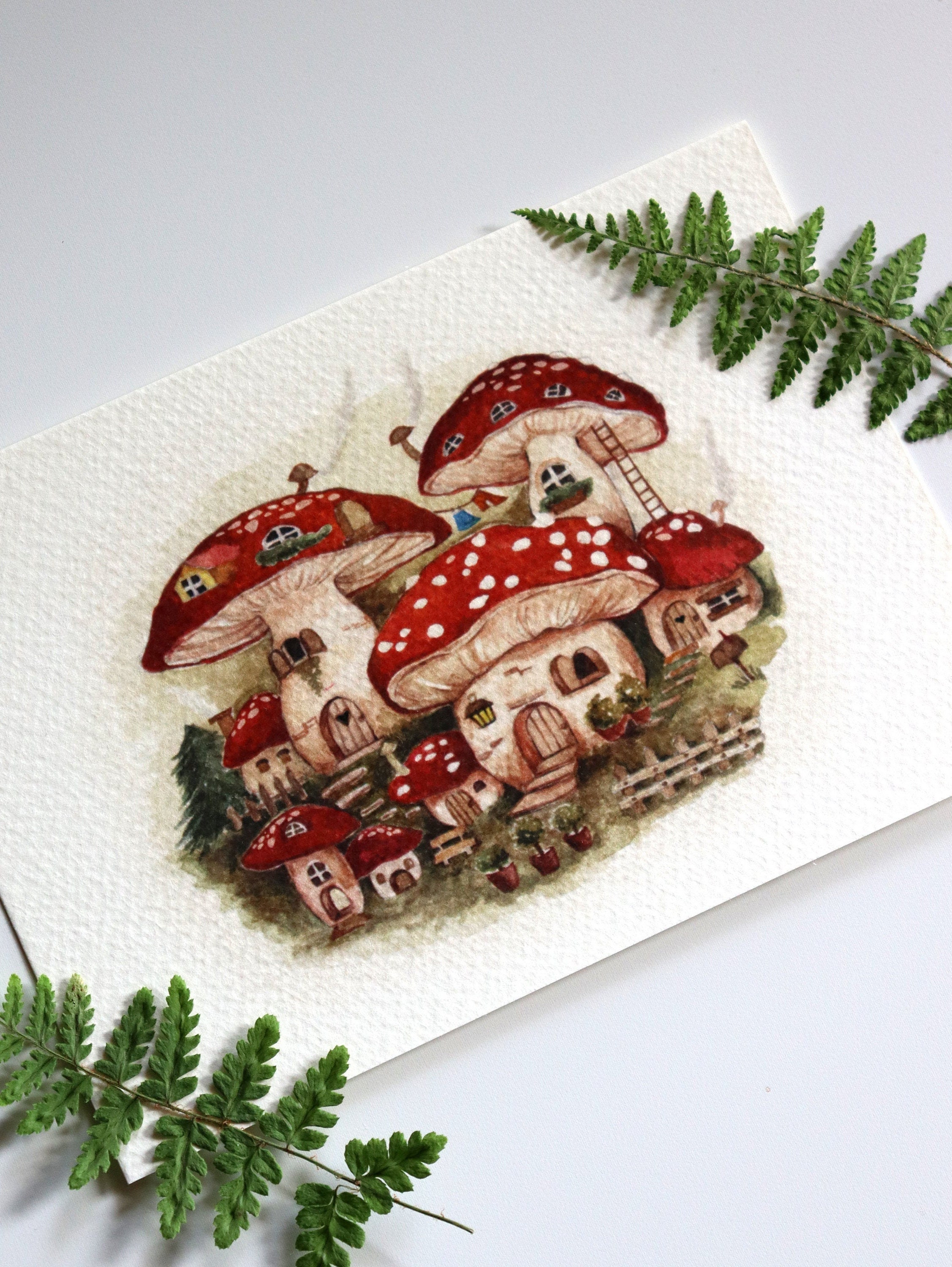This is a detailed color photograph of a textured watercolor postcard. The paper has noticeable ridging, suggesting a thick and sturdy cardstock-like material. On the light gray background of the postcard are two prominent green fern fronds, one positioned in the top right corner and the other in the bottom left. The central focus of the postcard painting is a whimsical scene featuring several mushrooms transformed into quaint houses. These mushroom houses have white stems and underparts, with vibrant red caps adorned with white polka dots. The houses are intricately designed with brown doors and windows, some featuring arched shapes. Ladders connect some of the mushrooms, and there are additional smaller mushrooms to the left, creating the impression of a playful, interconnected community. In front of the houses, there are small pots with plants and a white gated fence, adding to the charm. The postcard is slightly tilted, and it's apparent that the mushrooms are of varying heights and sizes, giving a dynamic, layered effect. There are also smokestacks visible on some of the mushroom houses, emphasizing their home-like appearance. Overall, the detailed illustration evokes a magical, somewhat animated feel.